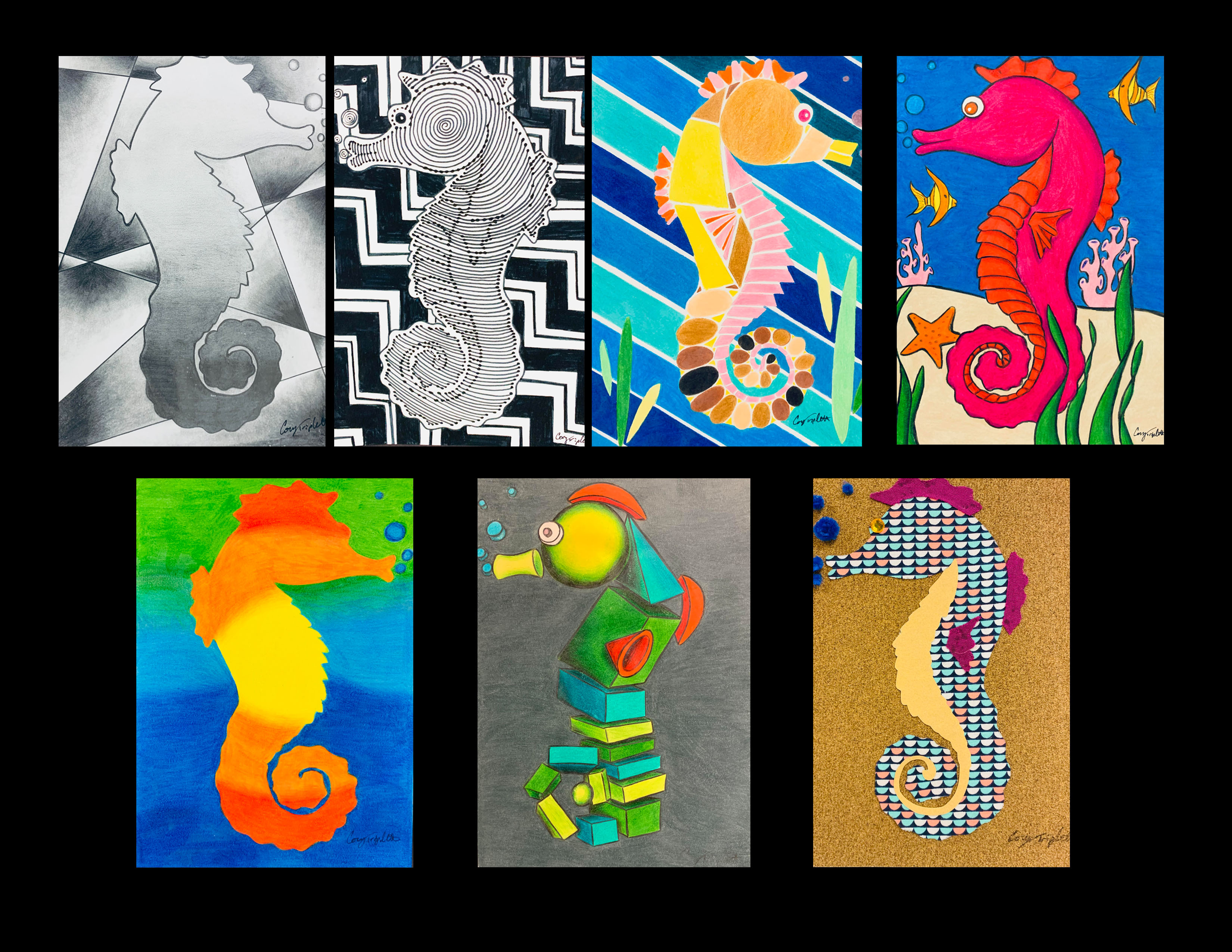The image features a black background with two rows of diverse seahorse illustrations, four on top and three on the bottom. Starting from the top left, the first seahorse is a black and white abstract, comprised of geometric triangles behind it. Adjacent to it is another black and white seahorse, surrounded by jagged shapes and swirling fingerprint patterns, accentuated with a black circular eye. Next is a vibrant seahorse set against a striped background of light blue, dark blue, and teal green, showcasing an orange, yellow, and red pastel palette. To the right, a seahorse painted in pink with orange accents inhabits an ocean scene with colorful fish, a starfish, and sandy seabed. On the bottom left, a tie-dye seahorse in shades of green, light blue, and darker blue faces right. Next, a robot-like seahorse with separate geometric shapes, including blocks and triangles in various colors, stands out against a gray background. Finally, a construction paper seahorse with a patterned body in light pink, blue, and darker pink, along with purple fins and a light brown belly, completes the lineup.